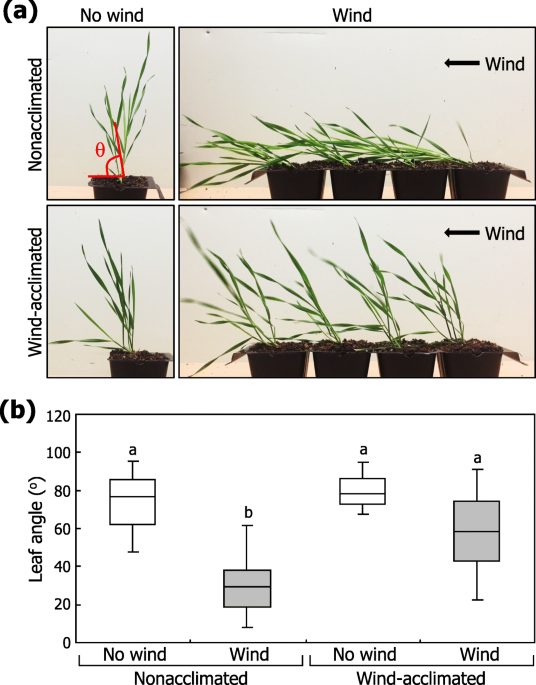This detailed scientific graphic illustrates the impact of wind on plants, highlighting how plants can acclimate to windy conditions. The upper portion, labeled "A," features four images arranged under categories: "No Wind" and "Wind," as well as "Non-Acclimated" and "Wind-Acclimated." It vividly depicts non-acclimated plants standing upright in no wind, but leaning heavily when wind is present. Conversely, the wind-acclimated plants show a slight lean in no wind and only a moderate additional tilt when exposed to wind, indicating their enhanced stability.

The lower diagram, labeled "B," provides a quantitative analysis of these observations. It focuses on the "Leaf Angle" and compares different conditions: "Non-Acclimated, No Wind," "Non-Acclimated, Wind," "Wind-Acclimated, No Wind," and "Wind-Acclimated, Wind." This graph quantifies the leaf angles under each condition, emphasizing the differences in plant behavior between those acclimated and non-acclimated to wind. Overall, the image effectively demonstrates the ability of plants to adapt and become more resilient to windy environments.